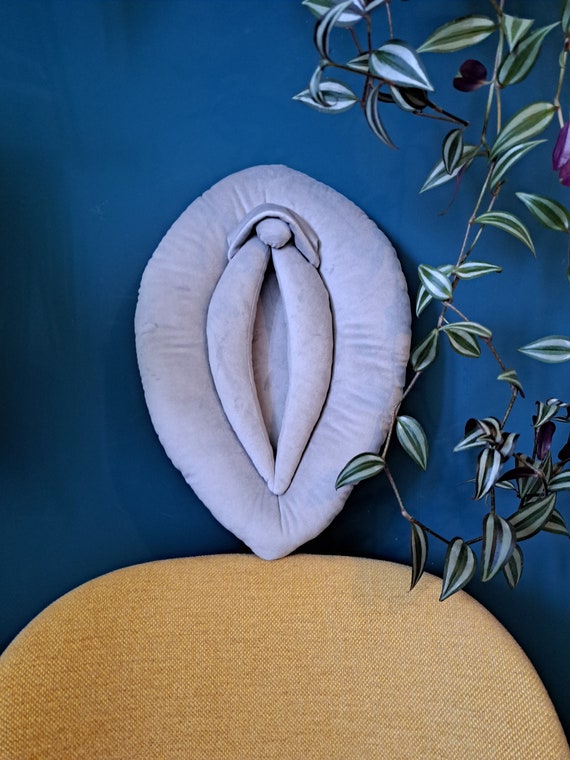A striking and eclectic household scene is captured in this image. Dominating the background is a deep blue wall, exuding a rich and calming presence. Centered against this vivid backdrop is a soft, yellowish-brown chair, reminiscent of golden wheat in color and texture. Suspended above the chair is an intriguing, pillow-like artwork in a bold shade of purple that contrasts sharply with the surrounding decor. Notably, the shape of this pillow is unconventional and thought-provoking. Adding a touch of nature, a vine-like plant with green and white leaves snakes its way through the scene, lending a sense of organic movement and life. Together, these elements create a vivid tableau of color and texture, showcasing an artistic and distinctive interior space.